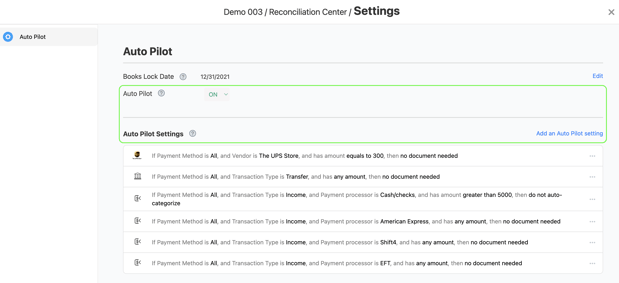Screenshot of a website interface depicting a subsection of a reconciliation center titled "Demo 003 / Reconciliation Center / Settings." The page has been accessed via a tab labeled "Autopilot" in the upper left corner. A prominent blue circular widget, likely representing a settings icon, is also present. 

The interface prominently displays the title "Autopilot," rendered in black text at the top. Below this, a section labeled "Book Lock Date" is visible, alongside a specific date. The page also includes options such as "Autopilot On" and "Autopilot Settings." Additionally, it provides detailed information concerning various payment methods and corresponding transactions, indicating whether the payments are incoming or outgoing.

At the top of the page, there is an "X" button in the top-right corner, presumably for closing the interface. Just above the section detailing descriptions and payment methods, there is a blue link labeled "Add an Autopilot Setting."